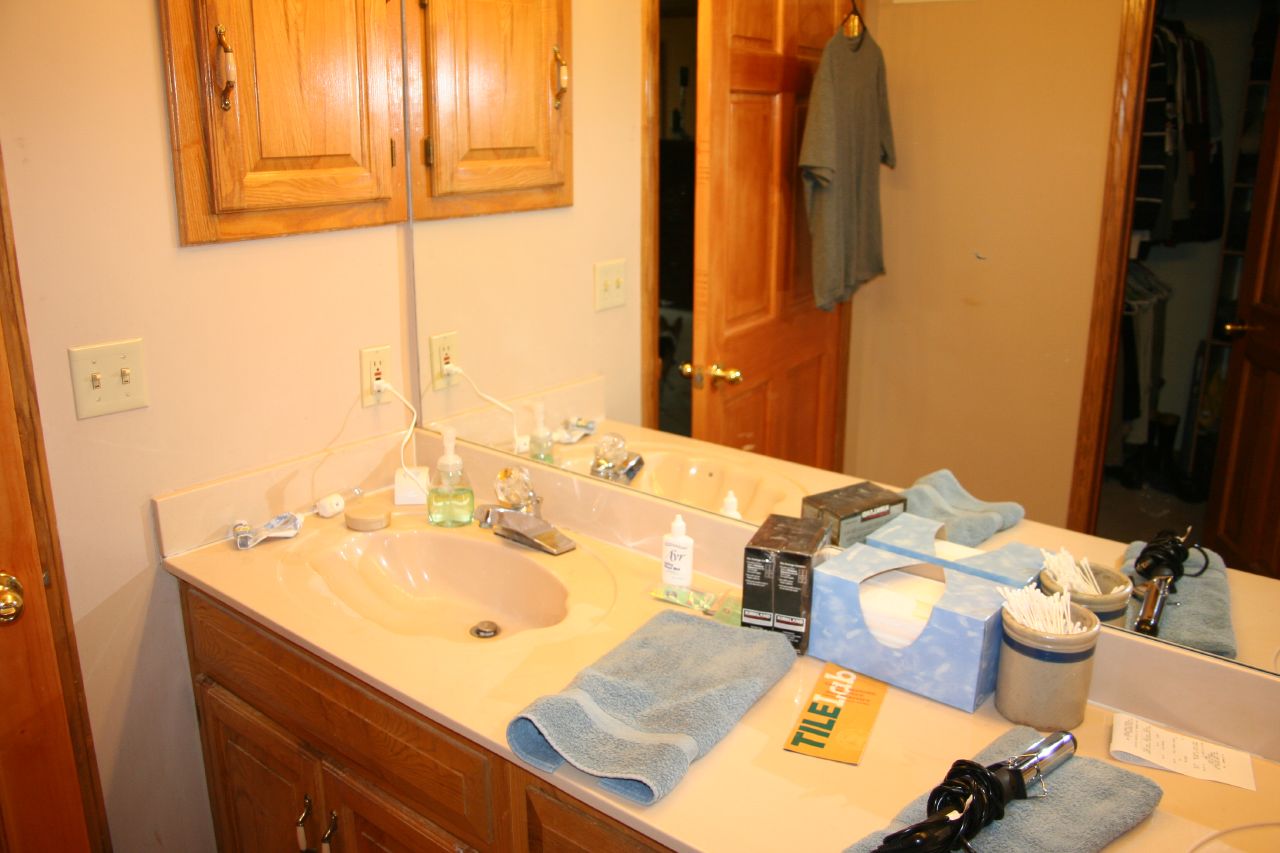This image captures the essence of a 1980s-style bathroom, rich with oak accents throughout. On the left side, there's a slightly ajar oak door featuring a brass handle. The door's reflection in a large mirror that spans the entire back wall reveals a gray t-shirt hanging behind it. In the mirror's reflection, there is another partially open door in the background, leading to what appears to be a bedroom, indicated by the glimpse of a bed.

Adjacent to the oak door, the wall is painted a light pink hue and is fitted with a double old-style light switch. Below the wall is a lengthy countertop made of a faux pink marble material with an integrated backsplash. This one-piece countertop features two built-in sinks, each adorned with chrome-plated faucets. Below the countertop, oak cabinetry provides storage space.

The countertop is topped with various typical bathroom essentials: a box of Kleenex, some towels, a hair curler, and other miscellaneous items, contributing to the lived-in feel of this nostalgic bathroom setting.